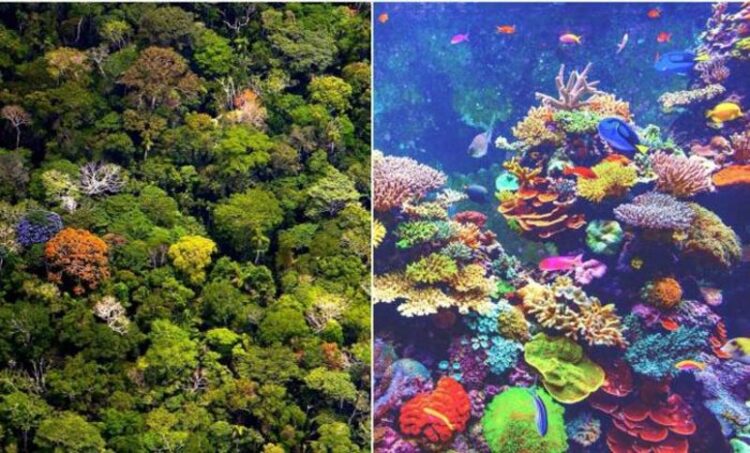The image displays two contrasting yet vibrant ecosystems side-by-side. On the left, an aerial view reveals a lush forest canopy dominated by varying shades of green, interspersed with sporadic bursts of lighter browns, and even an unusual purple hue. This mix of colors suggests a diverse array of tree species, creating a vivid and dynamic landscape. On the right, an underwater scene showcases a brilliantly colorful coral reef. The myriad of colors—ranging from greens, reds, and turquoise, to purples and blues—brings the reef to life. Tropical fish of various colors swim amidst the coral, adding to the scene's vibrancy, while the background, tinted in green and blue, features smaller, less distinct fish and more subdued coral forms. Despite some blurriness and distortion, the overall effect is a celebration of the rich and diverse beauty found in nature's different realms.